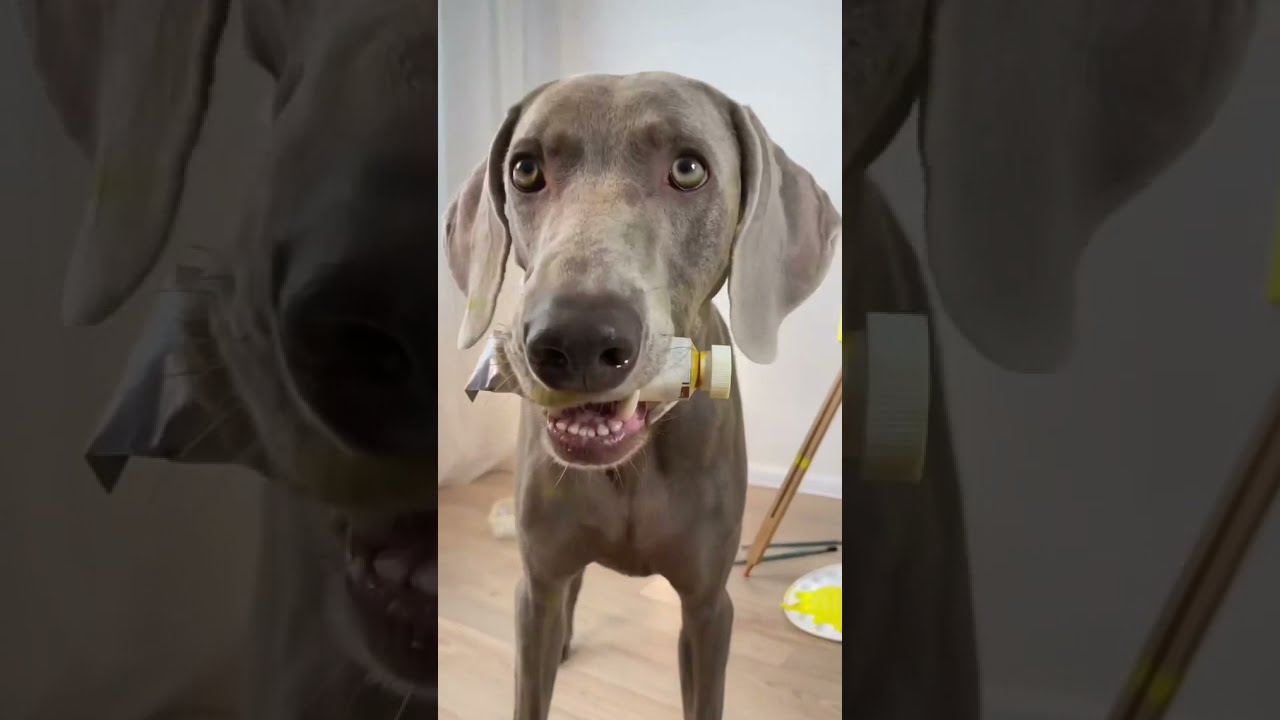The image features a thin, smooth-coated brown dog with floppy ears, light green (or hazel) eyes, a droopy expression, and a large, wet nose at the center. The dog is holding a tube of yellow paint with its cap still on in its mouth. The background showcases an enlarged, darkened version of the same image, creating a layered effect with the non-faded, more distant and detailed version of the image in the foreground. The dog stands on a light wooden floor. In the bottom right corner, there's a plate with yellow paint on it, likely serving as an artist's palette. Behind the dog, the legs of an easel are partially visible. The combination of these elements suggests a scene set in an artist's studio.